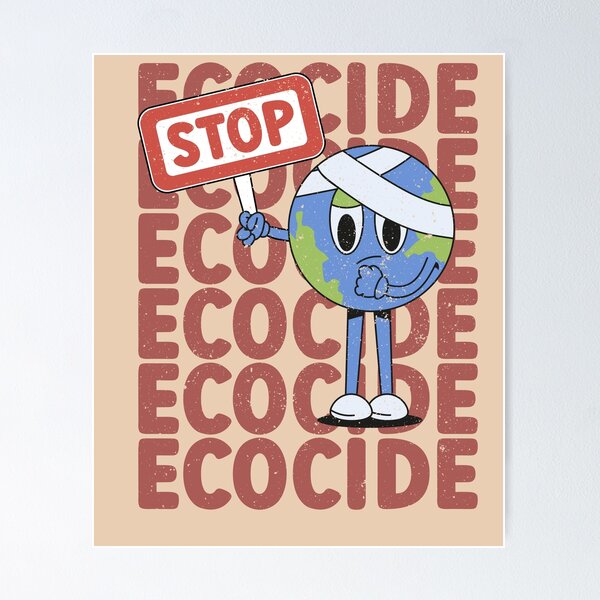This poster features a light tan background and prominently displays the word "ECOCIDE" in rust-colored, capital letters repeated six times in neat rows. In the foreground, there is a distressed cartoon representation of the Earth. The globe, illustrated with green continents and blue oceans, has elongated blue legs ending in white shoes. Its face shows large oval eyes with green eyelids and dilated pupils, adding to its expression of distress. The Earth character's left arm is held over its mouth in a gesture that suggests concern, and it has a white bandage wrapped diagonally across the top of its head. With its right arm extended to the side, the Earth holds a rectangular sign outlined in red, with the word "STOP" written in red letters on a white background. A small black shadow beneath its feet gives a subtle depth to the illustration. This poster conveys a clear message: "Stop Ecocide."